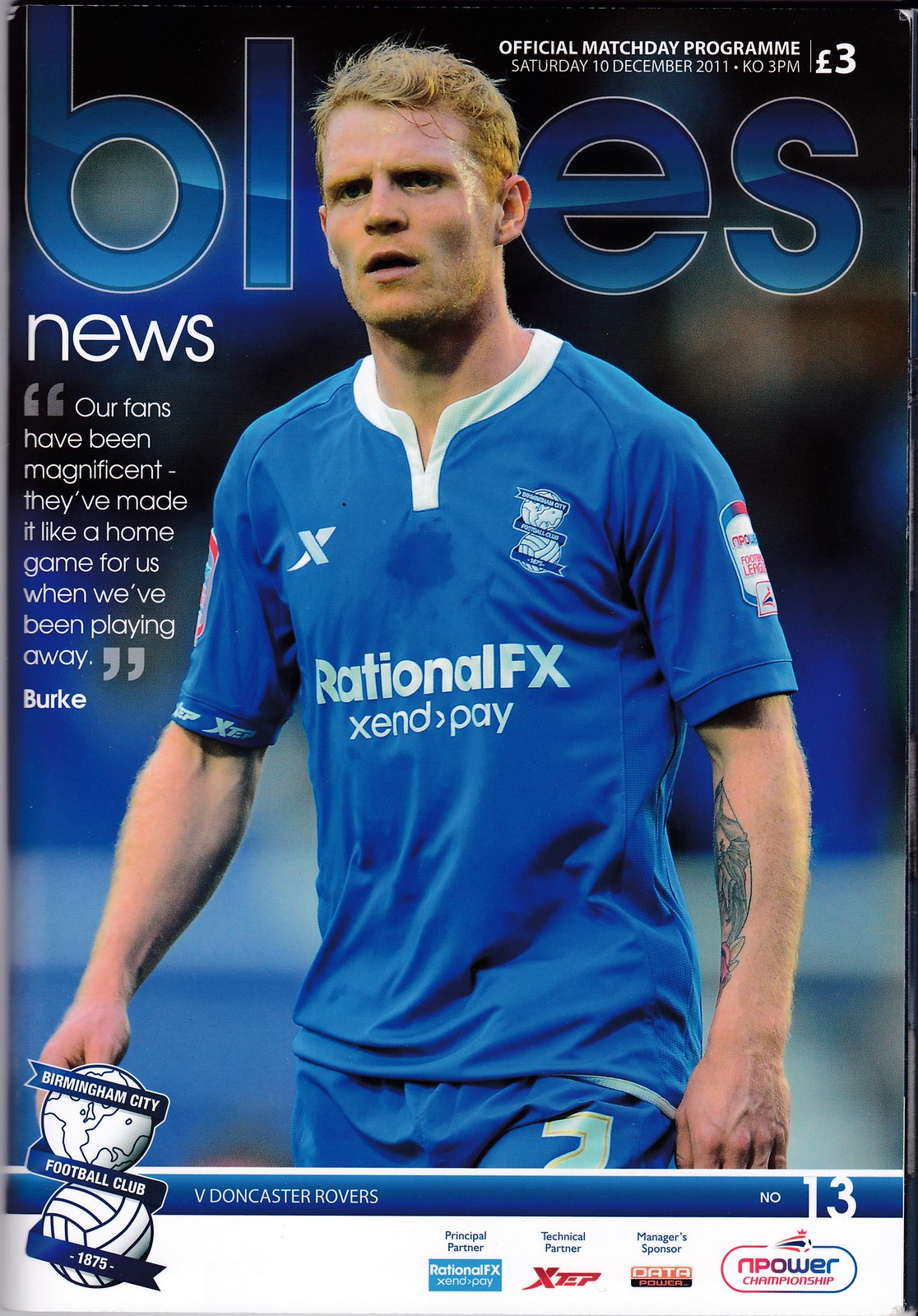This is a detailed magazine cover for a British football program, specifically for an official match day on Saturday, 10 December 2011, with kick-off at 3 p.m. Priced at three pounds, it features a striking image of a blonde football player in his thirties, dressed in a blue jersey with white collars and matching blue shorts. His uniform prominently displays the sponsor "Rational FX" on the front. Covering part of his face is the magazine's title "Blues," although the letter 'U' is obscured. The surrounding background is a blurred mix of blue and black hues. To the left of the player's image, white text reads "News," followed by a quote: "Our fans have been magnificent. They've made it like a home game for us when we're playing away," attributed to Burke. Above the title "Blues," it states "Official Match Day Program," along with match details against Doncaster Rovers. The top also includes the price of "£3," while the bottom right corner features the issue number "13" along with a list of sponsors.